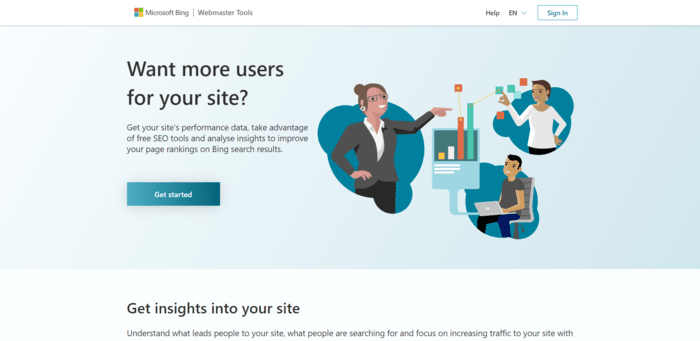This image is a detailed screenshot from a web page, specifically from Microsoft Bing Webmaster Tools. The header at the top has a white background, with the Microsoft logo on the left consisting of four colored squares—red, green, blue, and yellow. Next to the logo, the text reads "Microsoft Bing," followed by a vertical line, and then "Webmaster Tools" on the right. Further towards the right, there is a blue-outlined "Sign In" button.

The main section of the web page has a very light sky-blue background. On the left side, gray text reads, "Want more users for your site?" Below, it encourages users to, "Get your site's performance data, take advantage of free SEO tools, and analyze insights to improve your page rankings on Bing search results." Beneath this text, a medium-blue square button with white text says "Get Started."

To the right of the blue button, there are cartoon figures of three different people. The first is a woman with brown hair in a top knot, wearing a white shirt, a gray jacket, and dark brown pants. Next to her is another woman, light-skinned with brown hair, wearing a white long-sleeve shirt. Seated at a computer beneath them appears to be an Asian man with black hair, wearing a gray t-shirt.

At the bottom of the page, against a white background, the text reads, "Get insights into your site, understand what leads people to your site, what people are searching for, and focus on increasing traffic to your site with." The remaining text is cut off.